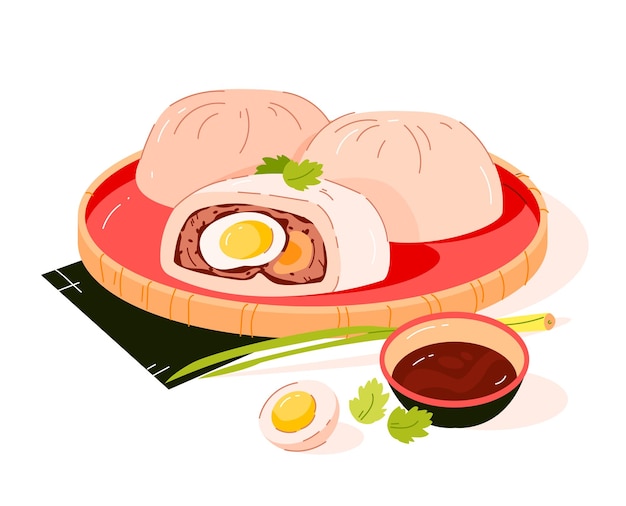This is a detailed cartoon illustration of three bao dumplings, also known as pork buns, arranged on a light wooden plate. The plate itself is bamboo with ceramic elements, featuring a pinkish hue with a tannish border highlighted by orange lines. Two of the buns are uncut and positioned behind a third bun, which is sliced open to reveal a filling of meat and a half-sliced hard-boiled egg. Accompanying the dish is a green parchment below the buns, a scallion placed in the foreground, and a condiment cup towards the bottom right. There is also an additional half-sliced hard-boiled egg to the right of the open bao. The arrangement includes various herbs on top of the buns, and the entire set is placed on a black platform with light tan shadows to the right, all set against a transparent background. The image has a high-quality, digitally-rendered, cartoonish art style.